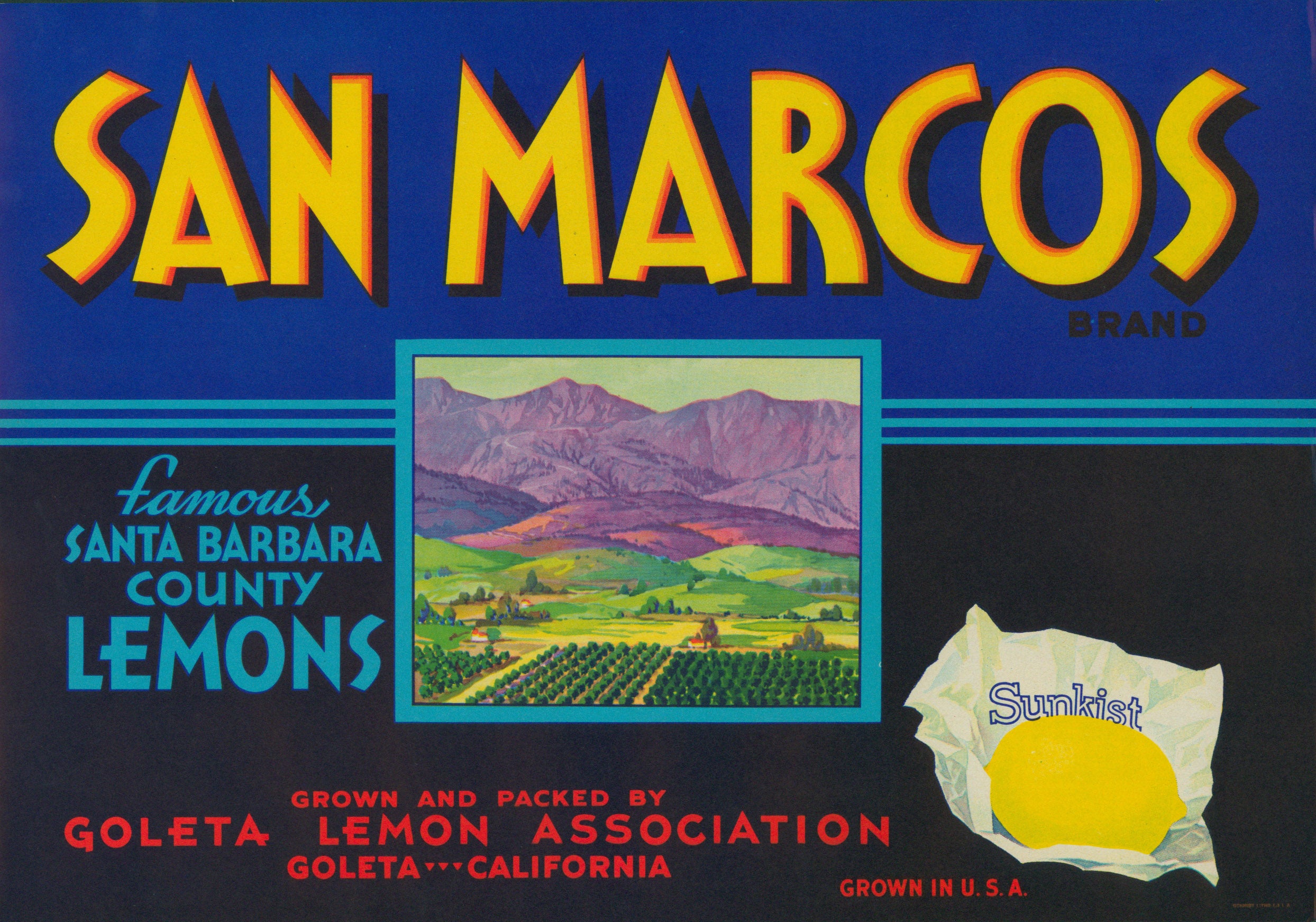This old-style advertisement for San Marcos brand features a vibrant and nostalgic design. The top half of the image showcases the title "San Marcos" in bold yellow text with orange trim against a blue background. Beneath it, the word "brand" appears in smaller black letters. The bottom half of the advertisement is set against a dark black background. Bold blue letters announce the product as "famous Santa Barbara County lemons." Centered in the lower half of the image is an illustrative scene depicting grassy hills, a farm, and a majestic mountain range in the backdrop, suggesting the picturesque landscape of San Marcos. Accentuating the local pride, red text reads, "grown and packed by Goleta Lemon Association, Goleta, California, grown in the USA." Finally, the bottom right corner features an image of a lemon wrapped in paper that is labeled "sun-kissed" in blue writing, adding a touch of authenticity and nostalgia to the advertisement.